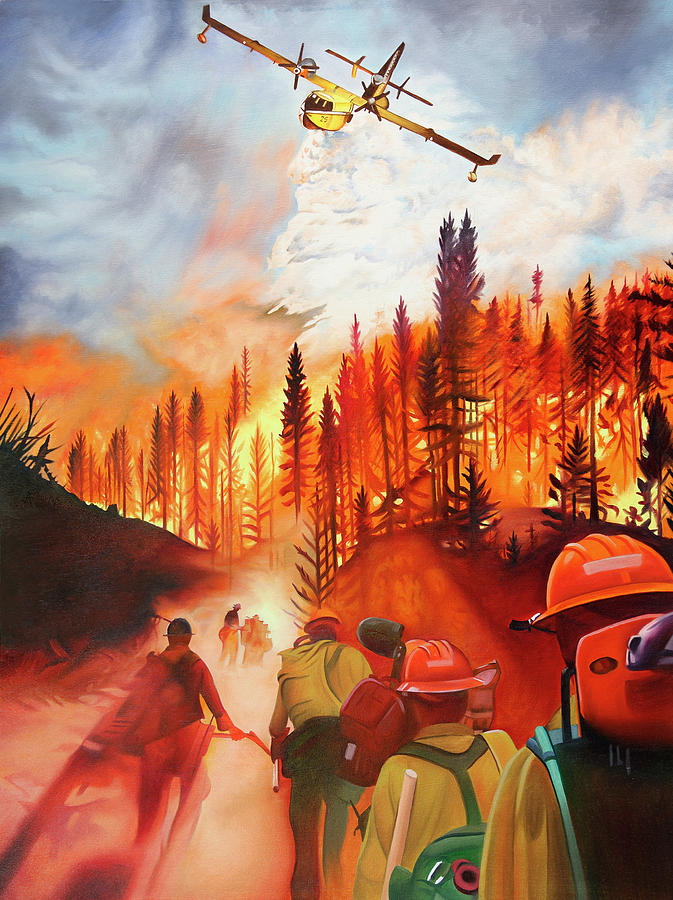This detailed and realistic painting depicts an intense forest fire with tall, skinny pine trees engulfed in vivid orange, red, and yellow flames. The scene is centered around this blazing inferno, with the ground appearing reddish from the intense heat and light. Above the fiery treetops, a yellow plane drops a white substance in an effort to contain the spreading blaze. Meanwhile, several firefighters, wearing helmets and equipped with packs, bags, and cans of water, are seen walking purposefully towards the heart of the fire, highlighted by a dramatic interplay of light. In the sky, above the smoldering treetops, there's a mix of smoke and clear blue sky, providing a stark contrast to the turmoil below.